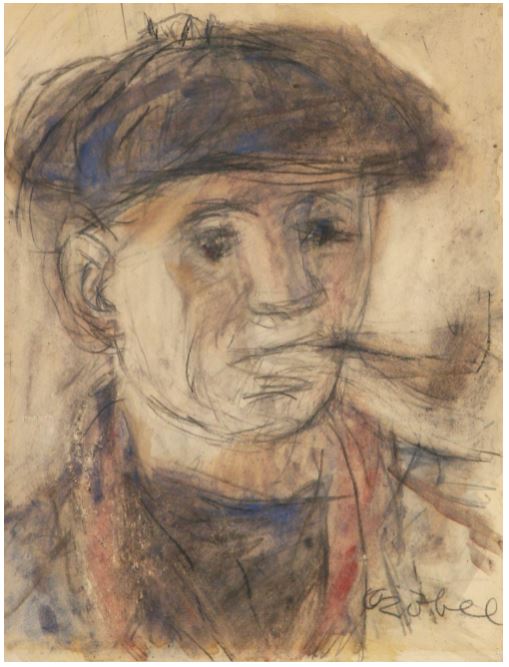The image depicts a loosely-sketched portrait of a man, seemingly a self-portrait, created using pencil or charcoal. The background features a blend of yellowish-gray tones, becoming darker around the shoulders and neck area. The man has prominent, dark eyes and a simple line forming his mouth, from which a brownish-red angled pipe extends. He appears to be wearing a newsboy cap or beret, characterized by its dark, almost oval shape. Draped around his neck is a deep red scarf or handkerchief, with traces of blue smudges blending into both the neck and head areas. The sketch's lines are intentionally messy and sketchy, with some sections painted over with watercolor hues. In the bottom right corner, there's an illegible signature. The overall composition includes subtle, stylistic smudges and strokes, adding depth to the portrait.